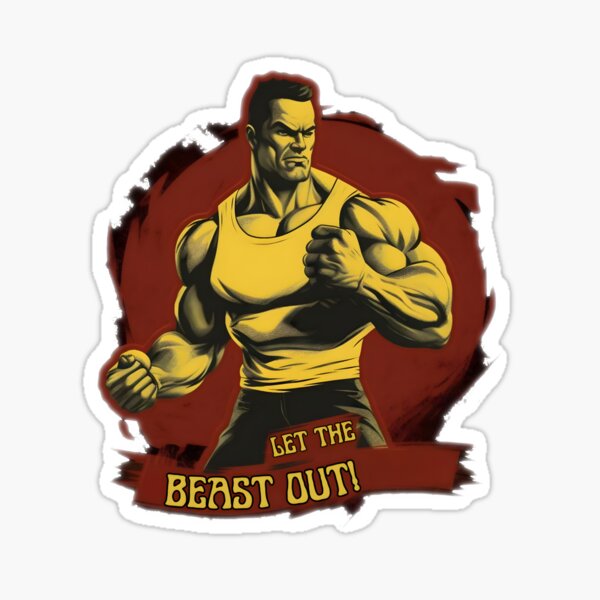This detailed image is of a die-cut sticker featuring an extremely muscular man set against a red or rust-colored circular background. The man, who has a yellowish-orange hue to his skin, is depicted with exaggerated, bulging muscles, particularly in his arms, chest, and shoulders. He is wearing a white tank top and tight black pants. His fists are clenched, with his left fist positioned near his chest and his right fist extended away from his body. His facial expression is intense and angry, with furrowed eyebrows and a grimaced mouth. The man has a short, closely cropped haircut. Below him, in pale yellow capital letters, is the phrase "LET THE BEAST OUT!" with an exclamation point. The overall aesthetic of the sticker gives a dynamic and aggressive impression, highlighting the man's imposing physique and fierce demeanor.